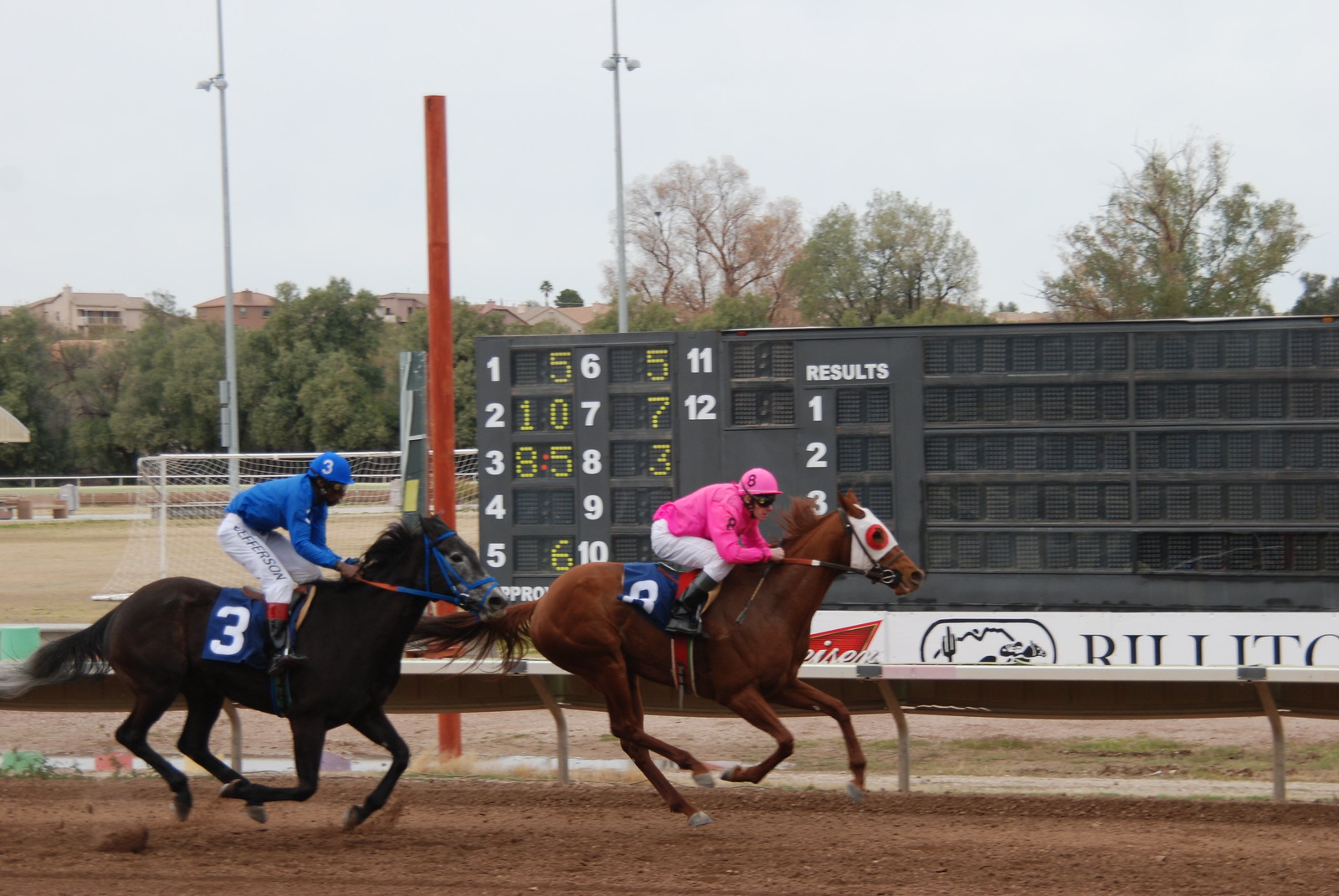The photograph captures a vibrant scene at a horse racetrack. In the forefront, two jockeys are racing their horses. On the left, a black horse with a gray face is adorned with blue stirrups and marked with a large number three on a blue flag attached to its saddle. Its jockey is dressed in white pants with black text on the side, a blue jersey, and a matching blue helmet featuring the number three in white on the side.

Beside them on the right, a brown horse with a distinctive white face mask accented by red circles around its eyes wears black stirrups. The jockey on this horse is clad in black riding boots, white pants, a pink long-sleeve shirt, and a helmet sporting a black number eight. A blue flag with a white number eight flutters from the saddle of the brown horse.

In the background, a lush field extends towards a goalpost, framed by a hillside dotted with several houses and trees. A prominent scoreboard displays the race results, highlighting the competitive nature of this horse racing event. The image vividly captures the intensity and excitement of the race, emphasizing the contrasting colors and details of the jockeys and their mounts.